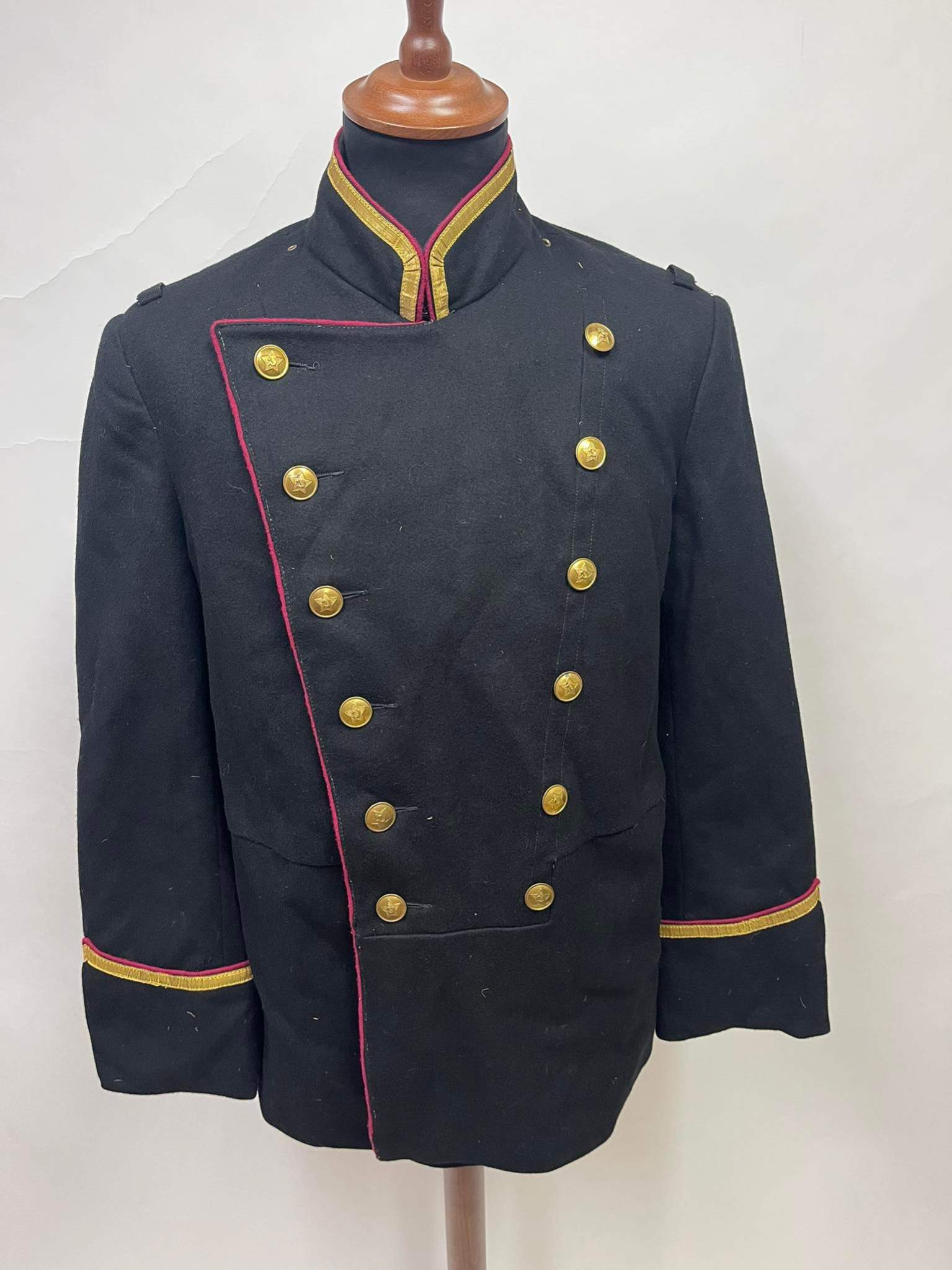The image depicts a historical military uniform, potentially from the Revolutionary era—possibly American or French, or even Civil War-period—displayed on a wooden stand that resembles a mannequin. The coat is primarily black or blue and features a prominent flap that buttons on the left side, with a total of twelve brass buttons—six on each side. The uniform is adorned with red trim running along the flap and gold fabric accents around the neck and cuffs, which extend partially down the sleeves and are outlined by red rings. The neck also features similar gold and red detailing. The brass buttons are intricately designed, potentially engraved with stars or eagles. The background includes a wall with visible cracks, suggesting that the uniform might be displayed in a museum setting.